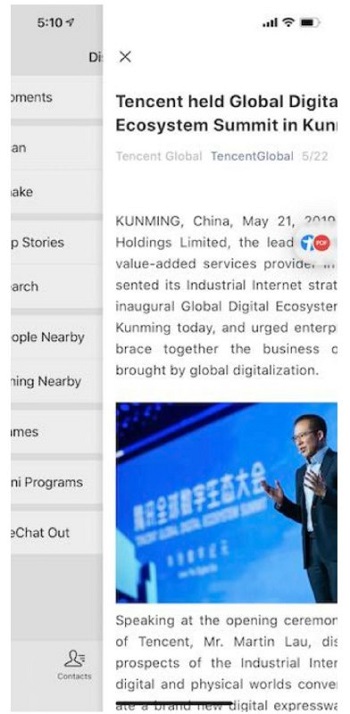A cropped screenshot from what appears to be a news reader app or an e-book reader app displays a partially obscured article and a navigation pane on the left. The navigation pane shows categories, including "Stories" and "Nearby Programs." On the right side, the article's title begins with “Tencent held global something ecosystem summit in,” but it’s cut off before completion. The visible part of the article continues with details like "Kunming, China, March 21st" and mentions "holdings, value-added" among other fragmented phrases. A highlighted section reads, “Speaking at the open, Tencent Mr. Martin Lau,” and this is paired with an image of Mr. Martin Lau at a venue. The image features a 40-something Asian man with glasses, standing in front of a crowd, with his hands raised in an expressive gesture. Behind him, a large screen displays Mandarin text on a blue background. The overall scene depicts a major corporate event but is presented in a way that leaves much to the viewer’s imagination due to the cropped view.